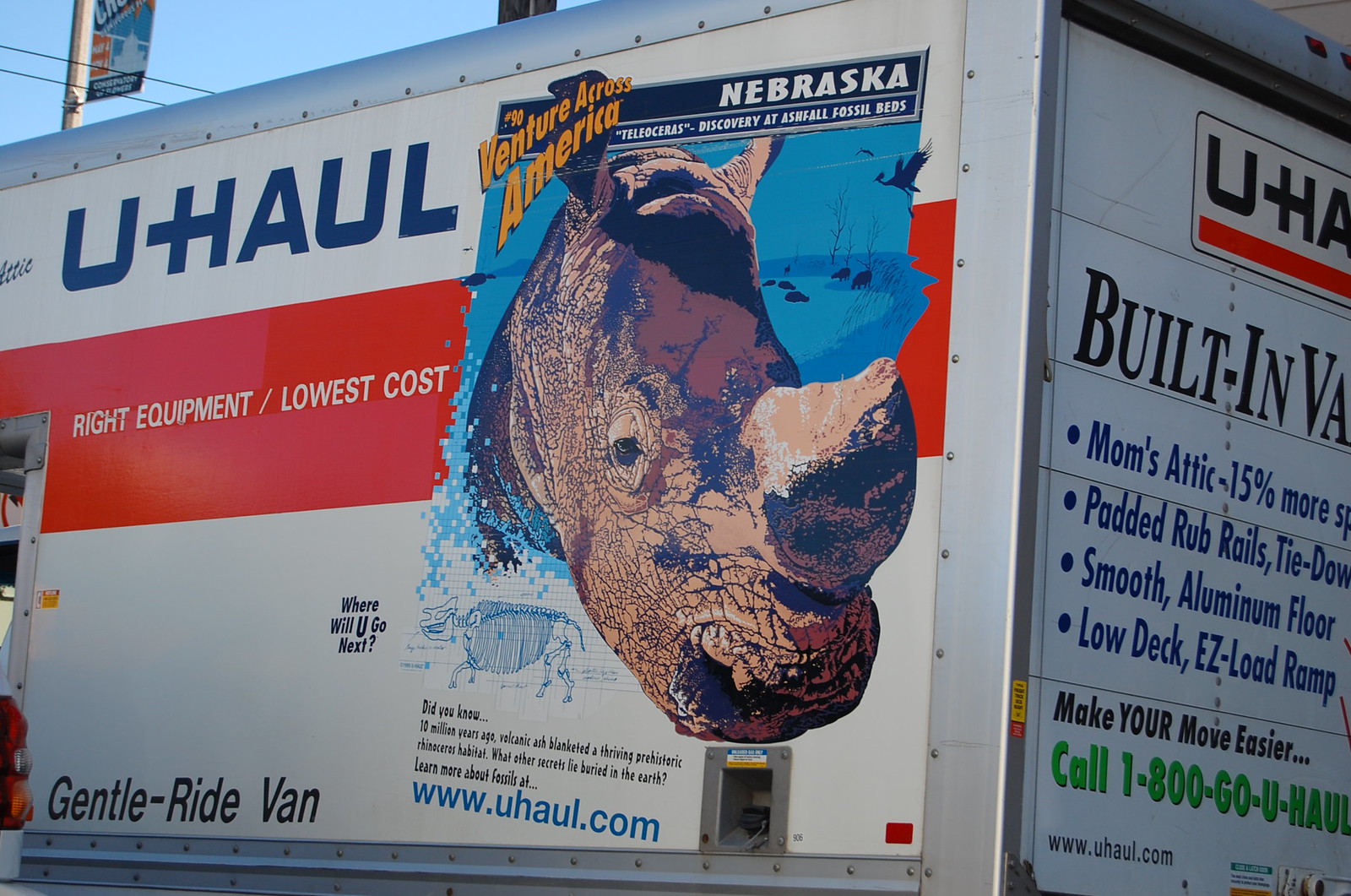This photograph captures a white U-Haul truck adorned with various informational and promotional graphics. Dominating the side of the truck, an orange banner displays the text, "Right equipment, lowest cost. Where will you go next? Gentle ride van." Prominently featured on the truck's side is an illustration of a rhinoceros, accompanied by educational text that reads, "Did you know ten million years ago, volcanic ash blanketed a thriving prehistoric rhinoceros habitat? What other secrets lie buried in the earth? Learn more about fossils at www.uhaul.com." This graphic also includes the title, "A venture across America, Nebraska, Teleoceras discovery at Ashfall Fossil Beds," indicating it is part of U-Haul's effort to share unique and intriguing facts about different states. The back of the truck offers a phone number for renting a U-Haul, further reinforcing its utility. The amalgamation of historical trivia with commercial messaging creates an engaging and informative visual experience, despite some confusion about the rhinoceros's relevance to U-Haul's primary services.